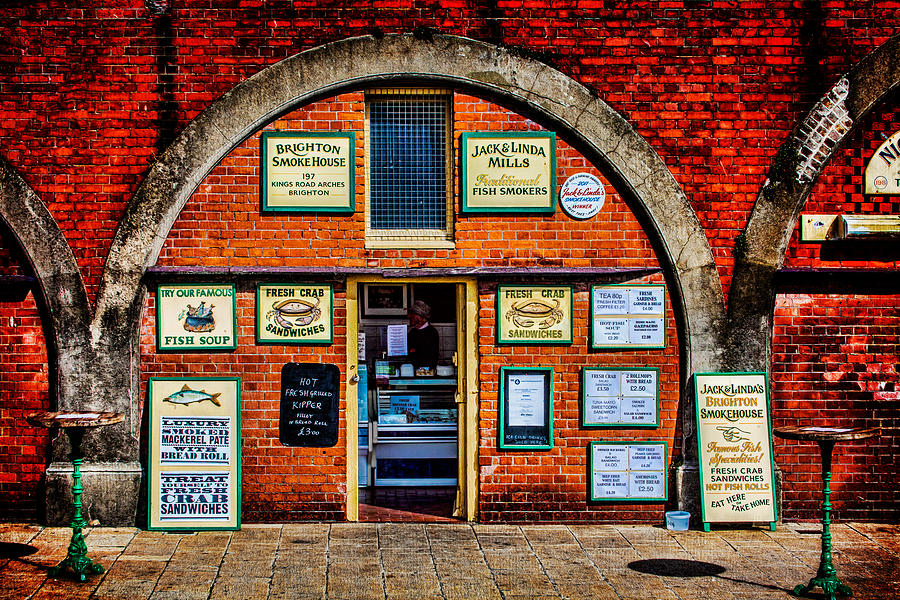The image depicts the bustling front of Brighton Smokehouse, a traditional fish market and deli housed in a charming red brick building. Dominating the storefront is a grand stone archway, topped with a green-boarded sign that reads "Brighton Smokehouse," flanked by multiple other signs promoting fresh seafood, including crabs and fish soup. To the right of the main arch is another green sign with green trim for "Jack and Linda Mills, Traditional Fish Smokers." The building itself is constructed with vivid red bricks outlined in white mortar, and a large rectangular window with a metal grate sits atop a door with a yellow frame, leading into the market where a man stands behind the deli counter visible through the propped-open door. Outdoor tables with green bases frame both ends of the storefront, adding to the market's welcoming atmosphere. The overall scene hints at a vibrant and inviting place with historical roots in seafood trade.